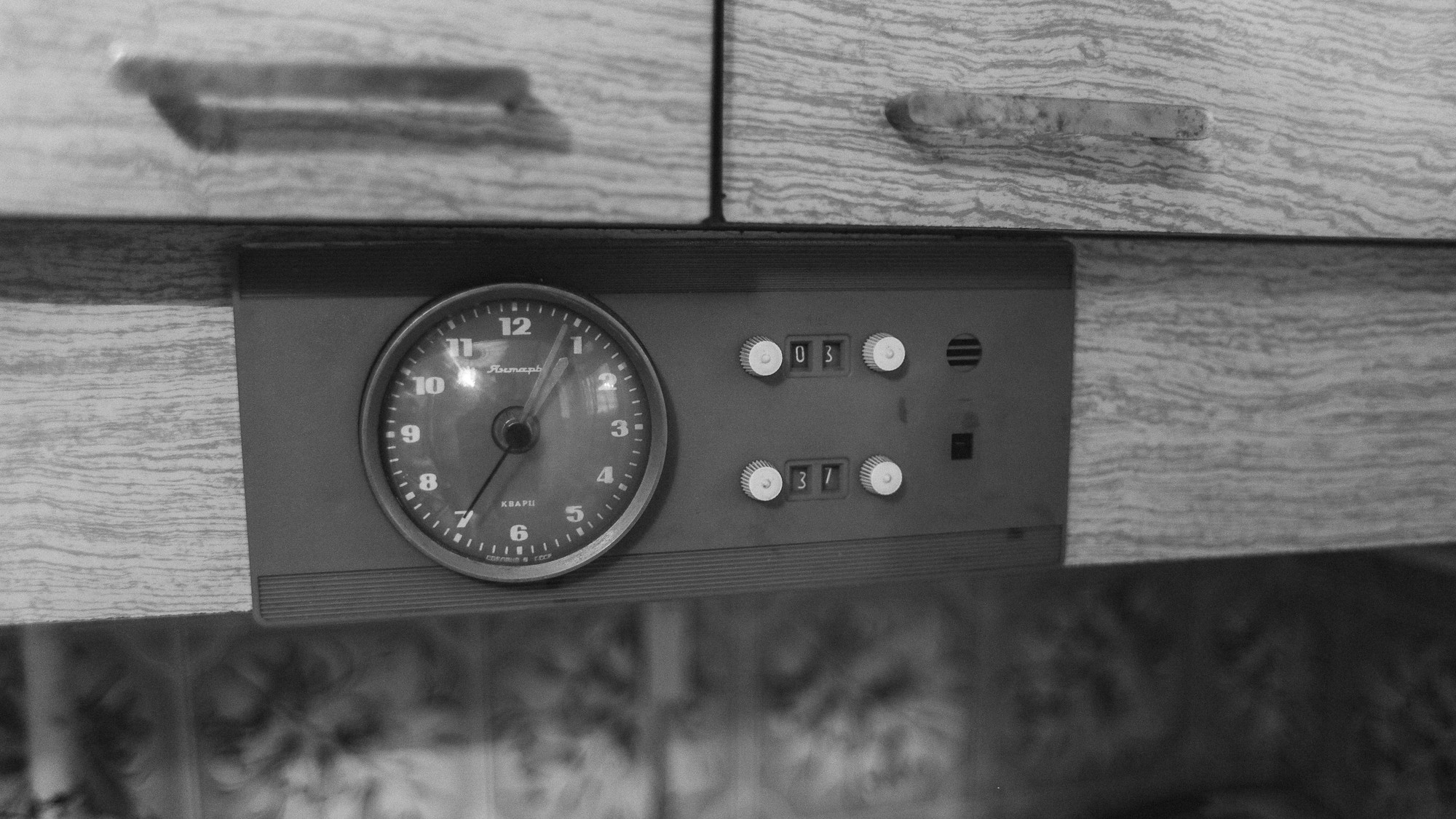This black and white photograph features a close-up of a distinctive clock embedded in a wooden structure, likely beneath a set of drawers or cabinets. The aged wood has vertical grain lines and appears slightly worn, accentuated by brass handles. The clock, housed in a dark gray or black rectangular casing, has a circular dial face situated on the left. The clock face is marked with numbers 1 through 12 and has minute markers, with bold dashes every 5 minutes. The time displayed is approximately 1:04, with the second hand pointing at the 35-second mark. To the right of the dial face are four white knobs arranged in a square pattern, each paired with number displays. The top display shows the number 03, while the bottom reads 37. The device also includes manual buttons flanking the number displays, used to adjust the digits. The entire scene is set against the backdrop of patterned wallpaper, adding a touch of vintage charm to the image.